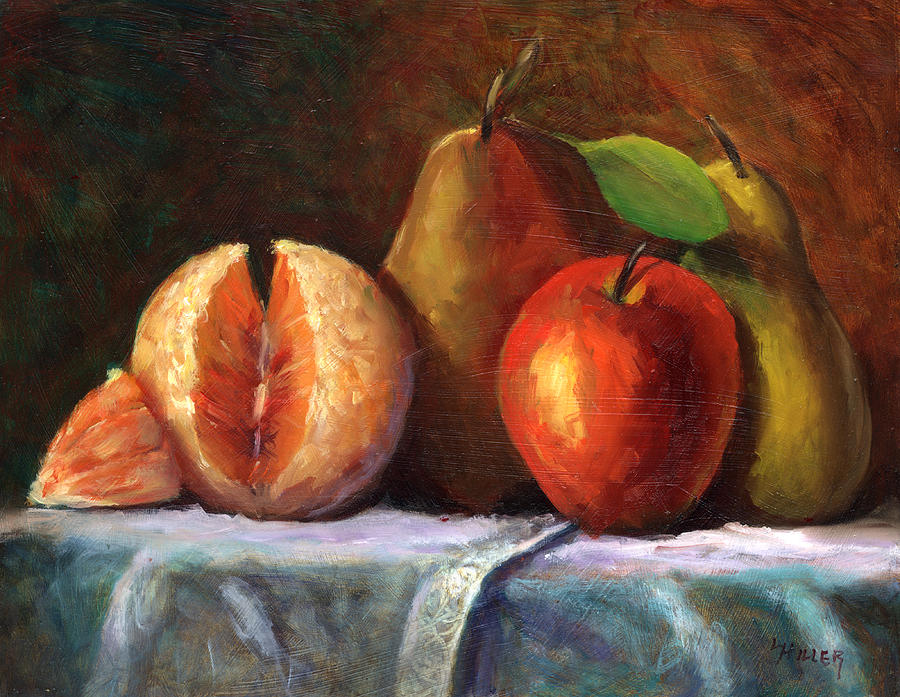This detailed still life painting portrays an arrangement of fruits set against a nuanced brown and red background. The gradient in the background shifts from darker tones on the left to lighter hues on the right, creating a subtle contrast with the vibrant colors of the fruit. The table they rest upon is draped in a white to off-white cloth, although some descriptions suggest hints of blue. The centerpiece is a bright red apple positioned prominently in the front. To its left, an orange rests, having been peeled with one segment placed beside it. Behind and to the right of the apple are two pears; the left pear is a darker shade of brown while the right one is more yellow. A closer inspection reveals a small detail, perhaps another piece of the orange or a small berry, near the orange. In the painting's bottom right corner, the artist's signature, "HILLER," is clearly visible in black capital letters. The overall composition of the fruits, along with the meticulous attention to color and detail, exemplifies the vintage charm of this artwork.